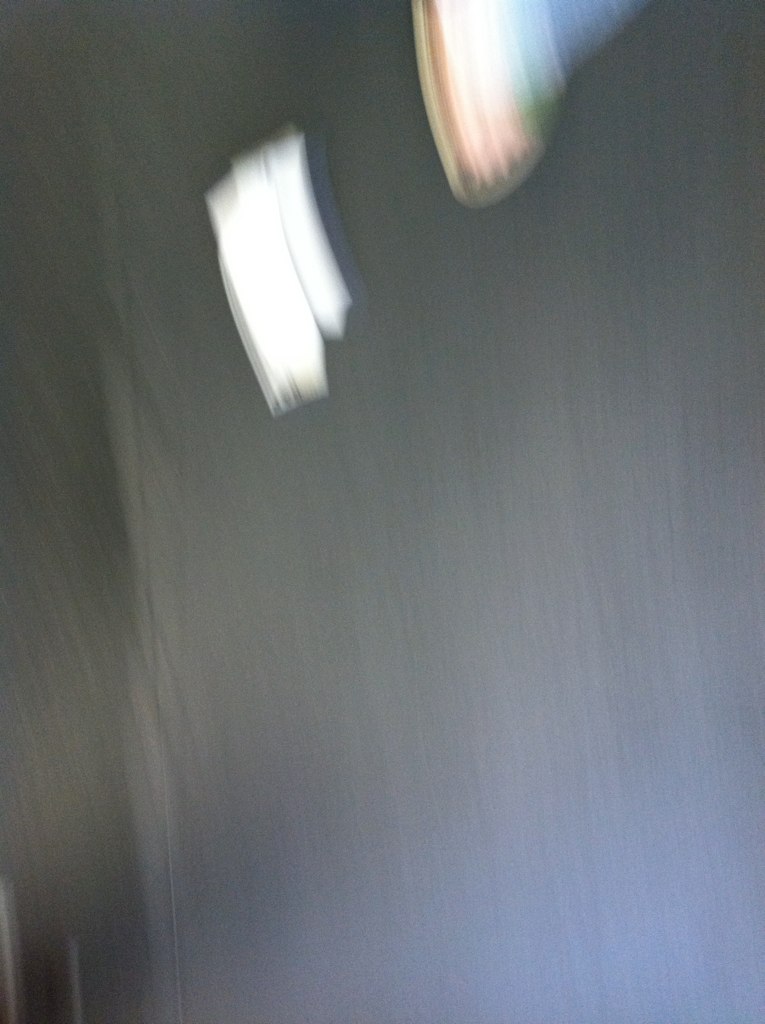A medium dark gray tablecloth serves as the backdrop for this image. In the foreground, a person's leg—adorned in blue jeans and a white shoe with red trim—extends towards the middle of the scene. There's a white, rectangular object situated centrally on the tablecloth, though its purpose remains unclear due to the blurriness of the image. At the bottom of the frame, two partially visible portraits are stacked one on top of the other, adding an intriguing yet obscured element to the composition.